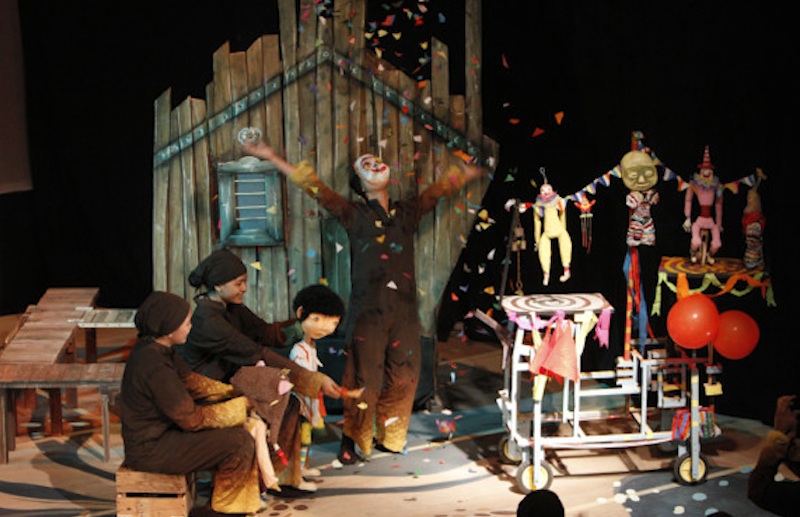This detailed image depicts a theatrical, almost surreal scene reminiscent of a cartoon like "Coraline." Central to the image is a figure, possibly a man or woman with a scarf-covered head, standing with arms outstretched towards the sky. They are surrounded by a shower of colorful confetti. To the right, several humanoid dolls and puppets, including a clown and an ogre, hang from strings attached to a wooden cart adorned with balloons and rags. 

To the left, two individuals, likely a woman and a young girl, sit passively on a small wooden bench. The girl is in a black head wrap, and the woman wears a black shirt and holds a Japanese-styled puppet. Behind them is a wooden prop house with a tiny window, reinforcing the theatrical or staged element of the setting.

Further details include a dark black background, stage lighting from below, and partial wooden walls with fixtures like an air conditioner. The entire scene blends elements of theatrical performance and surreal animation, with an undercurrent of spiritual or celebratory context underscored by the confetti and the character's reverent pose.